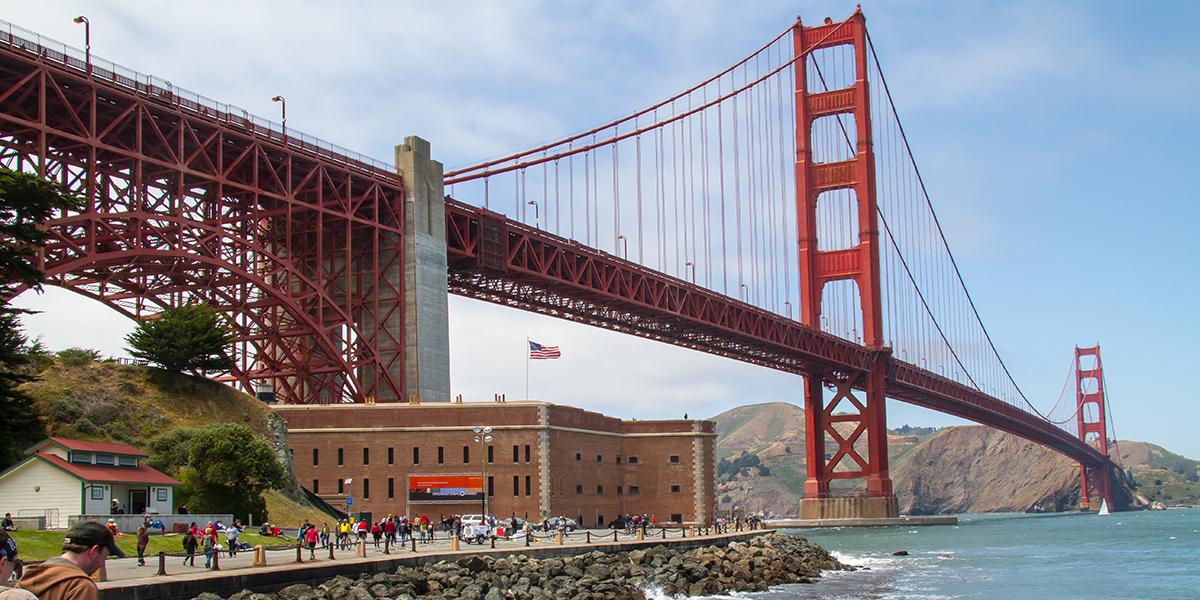This is a detailed photograph of the Golden Gate Bridge in San Francisco, captured on a bright, sunshiny day with a clear blue sky and faint, wispy white clouds. The iconic bridge, characterized by its dark red metal structure with lighter and brighter supports, extends diagonally from the top left to the bottom right corner of the image, spanning across a greenish-blue waterway.

In the foreground, on the left side, there is a bustling boardwalk with numerous people walking along it. The scene includes a prominent large red brick building, possibly a government or office building, with several windows and an American flag flying atop it. A small sign in front of this building displays red and black colors with blue writing.

Adjacent to the brick building, further left, is a smaller, white wooden building with an orangey red shingled roof. This building is perched on the edge of the San Francisco side, atop a hill covered with green grass and small trees or bushes. Towards the bottom left corner, a man wearing a baseball cap is seen looking down, while the surrounding walkway is dotted with indistinct figures of people.

In the background, across the water towards the bottom right, rugged brown mountains can be observed, adding to the grandeur of the photograph with their imposing presence.